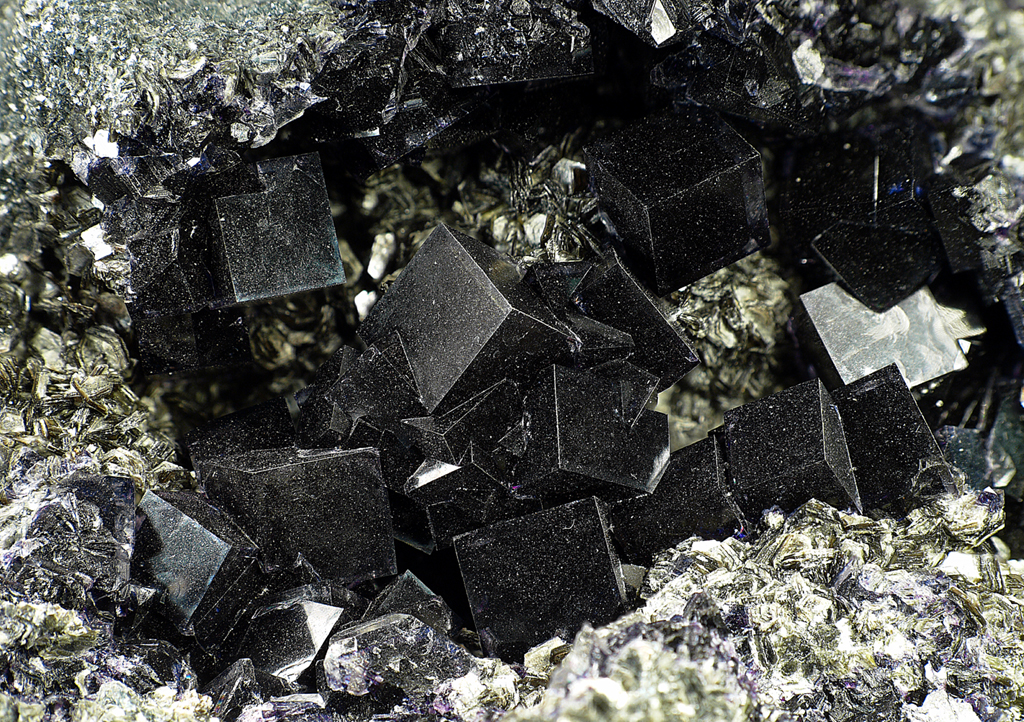The image features an intriguing array of black, opaque cubes, each with a glossy, almost obsidian-like surface. These cubes are interspersed with geometric shapes and positioned within a circular formation exhibiting a blend of gold and silver tones. The outer ring of the circle manifests a rugged yet smooth texture, reminiscent of natural rock formations. 

Within this circle, two prominent, glistening gold spheres command attention, surrounded by smaller, shiny black spheres scattered haphazardly. The black cubic forms appear randomly clumped together, with some morphing into triangular shapes. One cube is attached to a golden circular opening, while others seem to connect directly to the gold spheres, creating a striking contrast. 

A dozen or so of these cubes populate the image, their random distribution lending an air of natural authenticity. The lower section of the scene features a cluster of these shapes nestled together within a small recess, enhancing the overall complexity and visual intrigue of the composition.